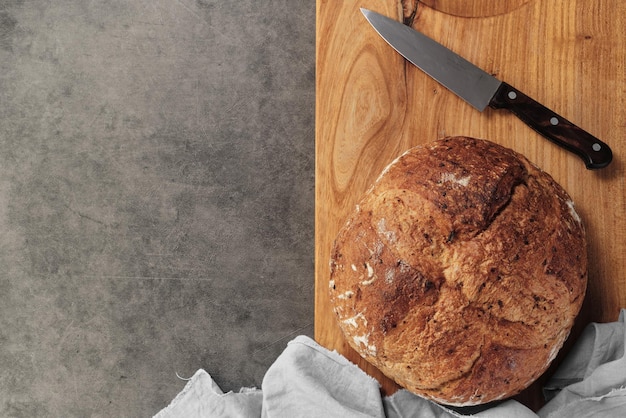The image depicts a neatly arranged culinary scene, potentially straight out of a magazine. Set on a varied gray marble countertop, a wooden cutting board with shades of brown offers a rustic touch. Dominating the board is a large, round loaf of bread, resembling sourdough, with a distinctive cross cut into its crispy brown crust, hinting at its fresh-baked nature. Dustings of flour cling lightly to its surface and base, adding to its artisanal charm. A sharp knife with a black handle and a gleaming silver serrated blade lies diagonally across the top part of the board, suggesting readiness to slice into the loaf. Below the bread, a white linen cloth gently wraps around its lower half, introducing a touch of softness to the arrangement. The colors in the image are predominantly neutral, with grays and browns harmonizing beautifully, emphasizing the simplicity and elegance of the scene.